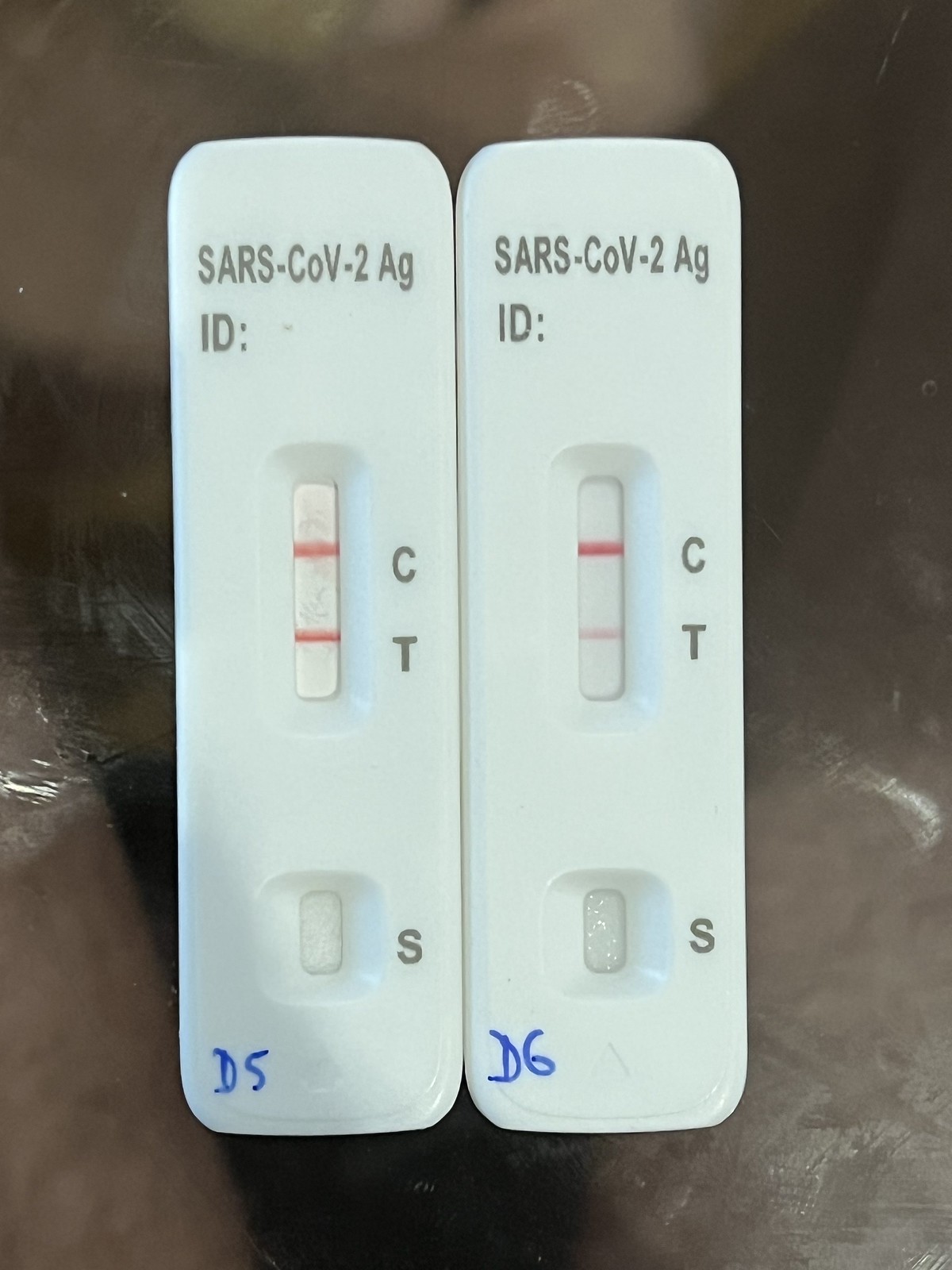In the image, we observe a vertically oriented composition with its height approximately 30-50% greater than its width. At the center of the image, there are two COVID-19 test kits positioned side by side, with the right edge of the left test kit touching the left edge of the right one. Each test kit is about four times as tall as it is wide and has an off-white color.

At the top of both test kits, black text reads "SARS-COV-2 AG" on the first line and "ID:" on the second line, with no further information following the colon. 

Centered on each test kit is a horizontal rectangular window displaying the test results. To the right of this window, the letters "C" (control) and "T" (test) appear in black lettering. The left test kit shows two red lines, one at "C" and one at "T," indicating a positive result, while the right test kit shows a solid red line at "C" and a faint red line at "T," indicating a possibly positive or inconclusive result. 

At the bottom of each test kit, there is a smaller vertical rectangle with a black "S" next to it. The lower left-hand corners of both tests are marked with blue ink: the left test kit is labeled "D5" and the right one "D6."